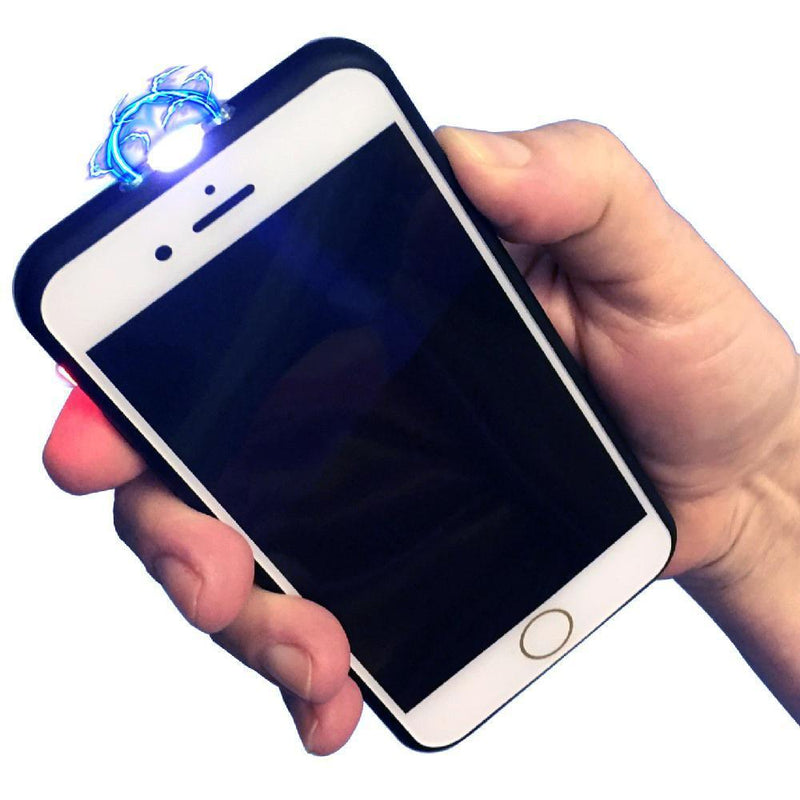The image depicts a white man's hand holding an older model iPhone, identifiable by its home button at the bottom of the device. The hand, visible from the wrist down to the palm, emerges from the right side of the frame and secures the phone by its sides, with all fingers visible on the far side and the thumb resting on one side. The white iPhone is encased in a black protective cover, which has distinct openings for the camera and microphone at the top. Overlaying the image is an eye-catching, blue lightning-like graphic that arches over the top of the phone, resembling a canopy. Additionally, there is a subtle red glow on the pointer finger, enhancing the surreal visual effect. The background has been edited to be a plain white, making the hand and the phone the central focus of the image.